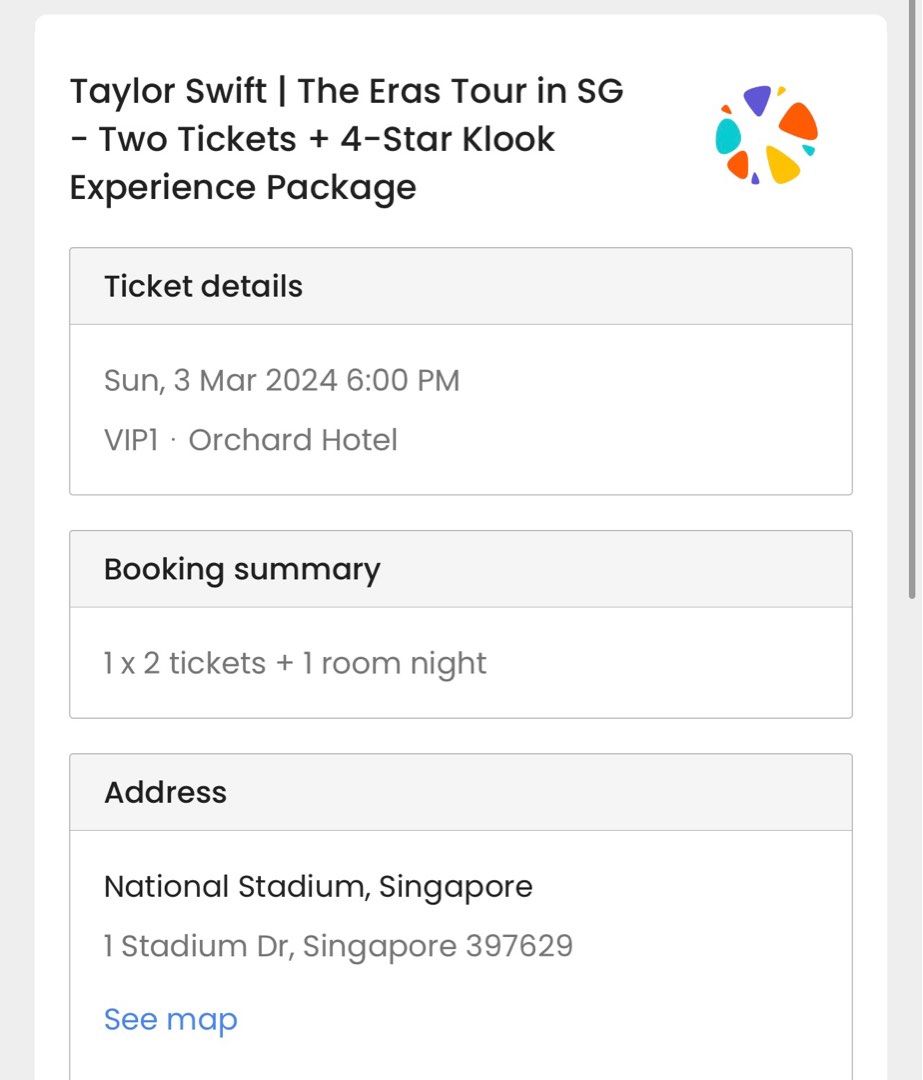This is a cropped screenshot of a concert ticket details page from a website or app. The image prominently features the information for a Taylor Swift concert, part of "The Arrows Tour," indicated at the top of the page. The user has purchased two tickets along with a "Four-Star Klook Experience" package.

On the top right, there is a round emoji adorned with triangular colorful blobs, adding a touch of visual flair. Below the title, a box labeled "Ticket Details" is visible on the left side, which outlines essential information such as the date, time, and seat location: Sunday, March 3, 2024, at 6:00 PM in VIP 1 section at Orchard Hotel.

Underneath, a "Booking Summary" indicates that the user has purchased a package consisting of two tickets and one room night. Further down, the address of the concert is provided: National Stadium, Singapore, complete with its full address. The bottom left corner features a "CMAP" hyperlink in blue text.

The screenshot also shows a vertical scroll bar on the right, positioned at the top, implying that additional information is available if scrolled down. The bottom of the screenshot is cropped, suggesting that more details lie beyond the visible portion of the page.